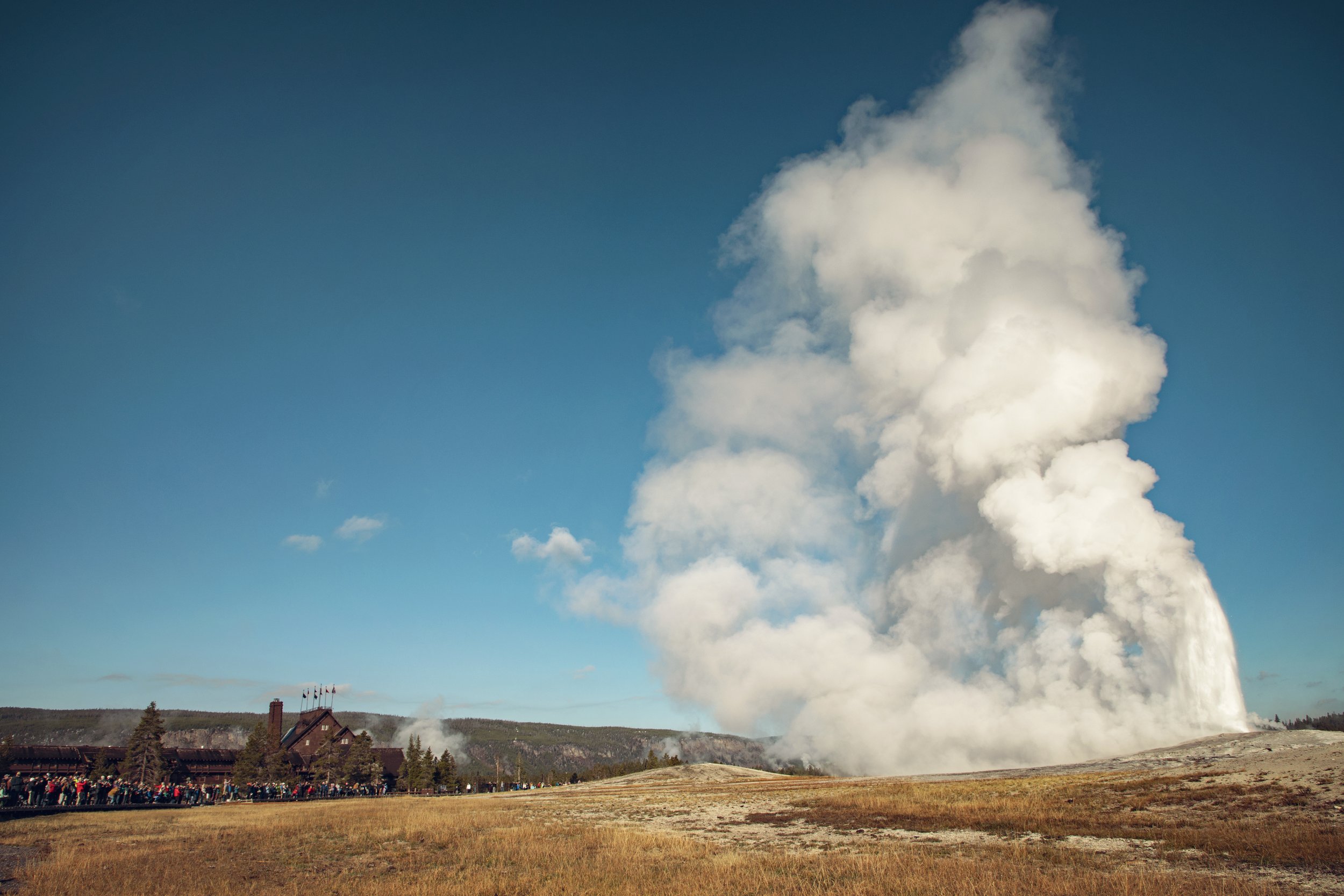The photograph captures a dramatic daytime eruption of the Old Faithful geyser at Yellowstone National Park in Wyoming, United States. Dominating the right side of the image, thick white steam ascends vigorously into a predominantly clear blue sky, slightly billowing outwards to the left. In the foreground and extending into the middle ground, a crowd of hundreds of tourists stand at a distance on a walkway, observing the geyser's impressive display. The scene is set against a contrasting landscape of hard-packed white dirt interspersed with patches of golden grasses. On the left side of the image, a large, rustic building, possibly the Hotel Yellowstone, features a peaked roof, a prominent chimney, and multiple flags. Further in the background, a series of gently sloping, green-capped hills rise, completing the picturesque setting of this iconic natural spectacle.